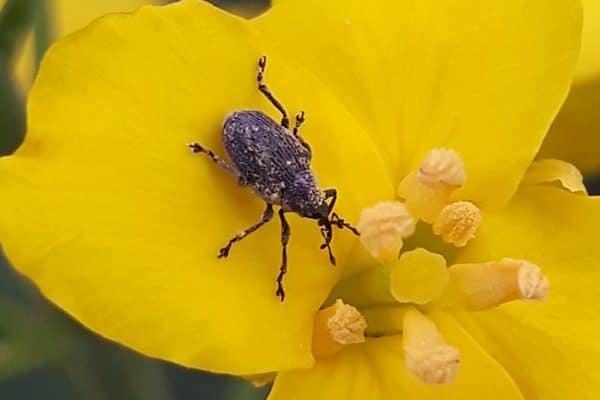This close-up macro photograph captures the intricate details of a vibrant yellow flower, focusing on about two-thirds of it. The flower boasts large, bright yellow petals with the visible top petal hosting a distinct insect. The center of the flower, located towards the bottom right of the image, reveals several yellow pistils emerging from it. The insect, resembling a beetle, is perched on the upper left petal. The beetle features an oval body with a predominantly brown and black coloration, and a black head. It has six legs, two antennae, and appears dusted with pollen. The beetle is positioned to face downward, seemingly toward the flower's center. The background showcases a beautifully blurred blend of light and dark green shades, allowing the vivid details of the flower and the beetle to stand out prominently.